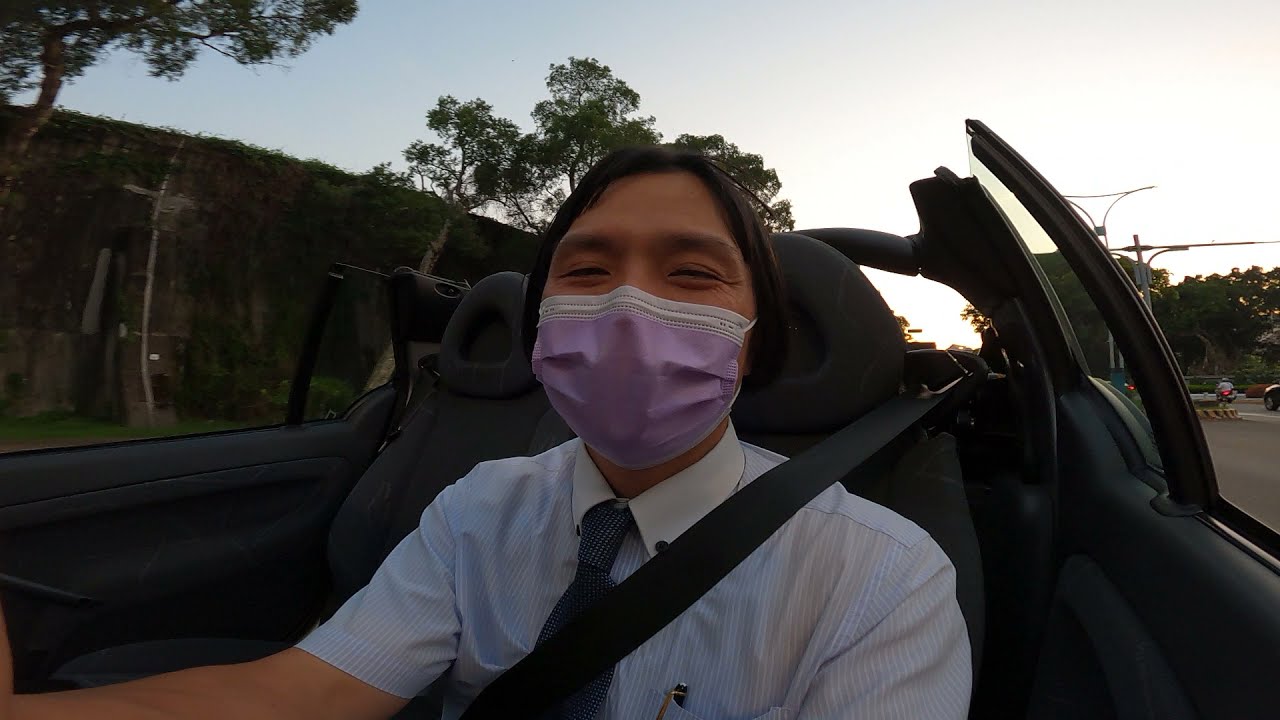This vibrant photograph depicts a man of Asian complexion, seated in the driver's seat of a black interior convertible car, characterized by its missing roof. The man is dressed in a white short-sleeve button-down shirt, accessorized with a grey tie adorned with white dots, and is wearing a purple mask that conceals most of his facial expressions. However, the slight crinkling of his eyes suggests a smile. He is securely fastened with a seatbelt and has a pen tucked in his shirt pocket. One can also see his right hand and elbow extended, indicating he might be handling the steering wheel. The car's interior contrasts sharply with the bright, clear blue sky above. Surrounding the car, the landscape features several trees and a cliff-like area with grass and dirt on the left. In the background, there's also a road with some vehicles and tall street lighting poles. To the far right, there appears to be someone on a bicycle, further enriching the scene with dynamic elements of everyday life.